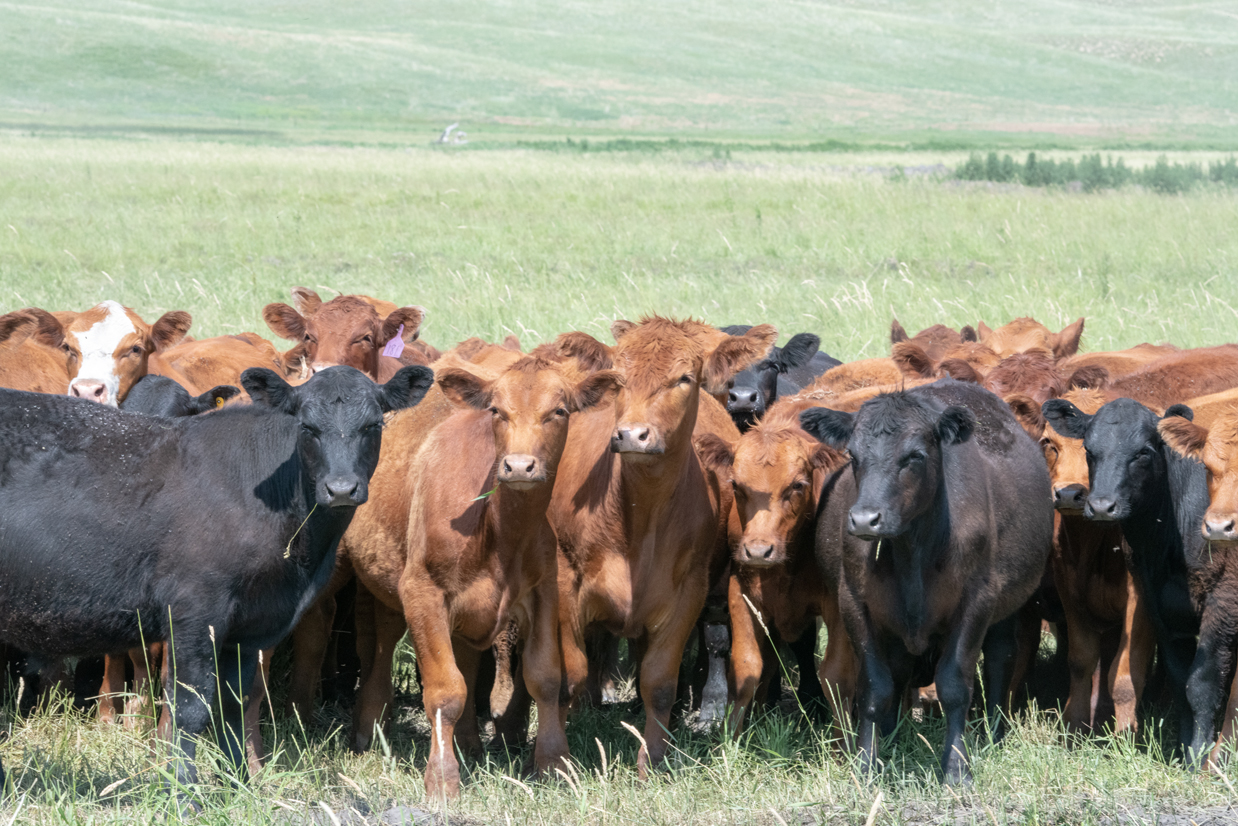This landscape-oriented color photograph captures a close-up view of a densely packed herd of cows, predominantly positioned in the lower half of the frame. The cows, a mix of black and light brick red, stand so close together that they are touching, their bodies forming a tight-knit group. On the left side of the image, a cow's body is turned to the right with its head looking back towards the viewer. The other cows, primarily facing forward, add to the cohesive gaze directed at the camera. No horns are visible on any of the cows, and their plump frames suggest good health, with a couple of them having pieces of grass hanging from their noses. The ground beneath their hooves is covered in a small strip of green grass, extending into a broad, grassy expanse that continues into the distance. On the right side of the background, a stand of trees provides a contrast to the grassy field, beyond which lies a hillside covered in verdant grass that slopes upwards and away from the viewer. The image exemplifies photographic realism, capturing the serene yet attentive presence of the cows in their pastoral setting.